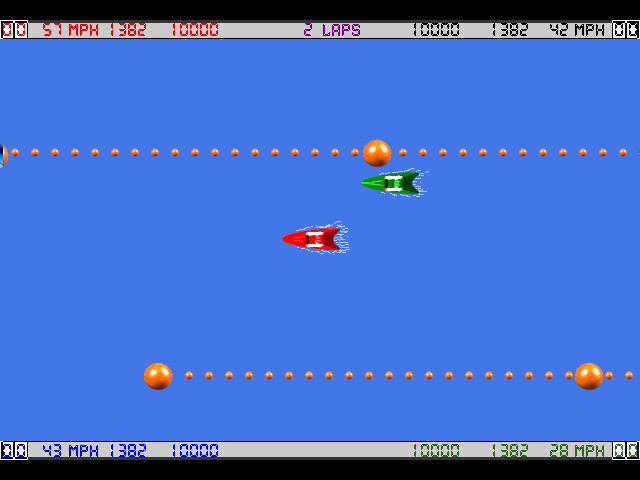The image is a detailed screenshot from a retro-style racing video game. The background is a cauliflower-blue color with two triangular shapes in the center, representing boats or spaceships. The red boat is positioned in front of the green one. Both shapes have small white lines extending backward and are surrounded by dotted sequences of orange lines and larger dots extending to the left and right. 

The top and bottom of the screen feature black borders containing various game details, including scores and speed indicators. The top of the screen shows "57 MPH" in red, "2 laps" in purple, and various numbers such as "10,000," "1," "3," "8," and "2" arranged in black and white squares. Similarly, the bottom of the screen displays "43 MPH" in blue and a similar array of numbers. Additionally, there's a gray rectangle with the legend "00" and respective indicators for miles per hour (MPH), presumably for each player. 

The image suggests an ongoing race, with the two boats, represented by geometric shapes, navigating across the screen in a competitive setup. The dots and lines interspersed with larger circles seem to indicate the track or a form of boundary/guideline for the race. Overall, it vividly captures the essence of a vintage racing game with vibrant colors, clear indicators, and a competitive atmosphere.